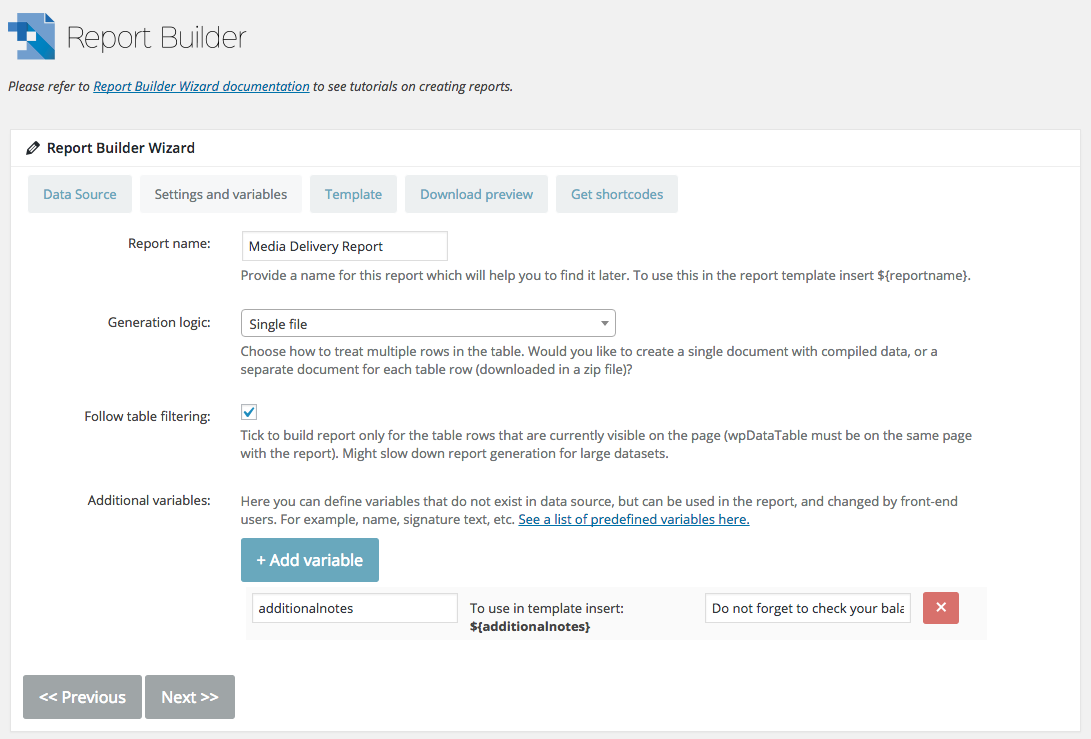In the image, at the top left, the title "Report Builder" is prominently displayed next to a logo resembling a piece of paper with a pixelated section cut out. Just below this, there is a note saying, "Please refer to Report Builder Wizard Documentation to see tutorials on creating reports," with "Report Builder Wizard Documentation" highlighted in blue and underlined. Beneath this note, the phrase "Report Builder Wizard" appears again in black text, accompanied by a small pencil icon to its left. 

The main section of the image is divided into five categories: "Data Source," "Settings and Variables," "Template," "Download Preview," and "Get Shortcodes." 

On the far left side, additional labels and options are visible, including "Report Name," "Generation Logic," "Follow Table Filtering," and "Additional Variables."

At the bottom right corner of the image, a small square box with a white "X" on a red background is noticeable. To its left, there is a rectangular notification area with the reminder, "Do not forget to check your bell."

The overall layout and design of the image appear to be part of a user interface for a report-building tool, with clearly defined sections and helpful documentation links.